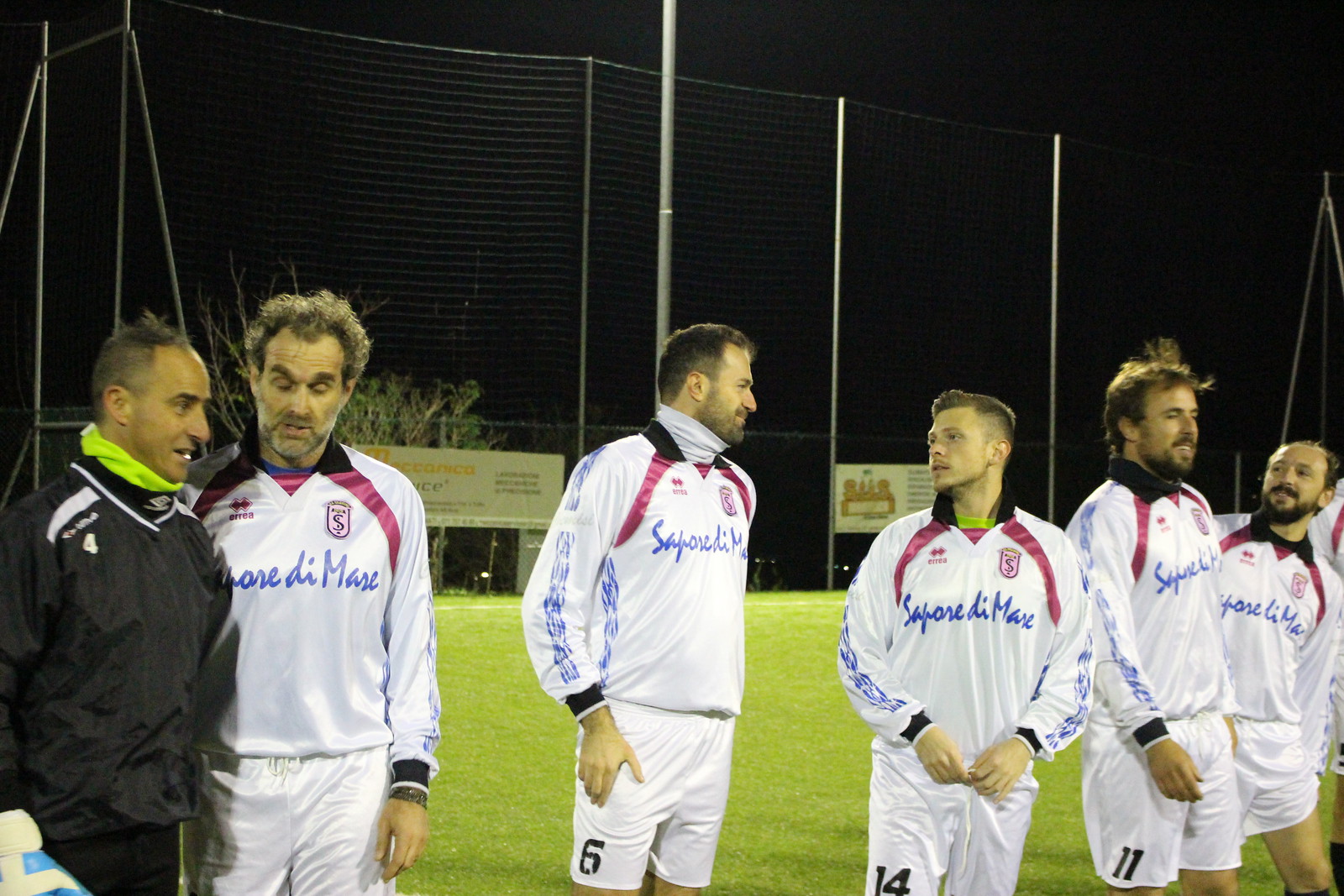In this nighttime photograph, a group of six men, likely a soccer team, is standing on a well-lit sporting field with green grass. Five players are wearing matching uniforms consisting of white long-sleeved shirts with red stripes running under their arms, and white shorts, some of which display numbers: 6, 14, and 11. The sixth man, likely the coach, stands to the far left, distinct in his all-black attire. The players appear to be conversing, with three of them sporting close-cropped beards while one in the center is clean-shaven. Behind the group, a tall fence adorned with banners encircles the field, illuminated by the field lights, with a glimpse of greenery, possibly strawberry plants, visible beyond the fence.